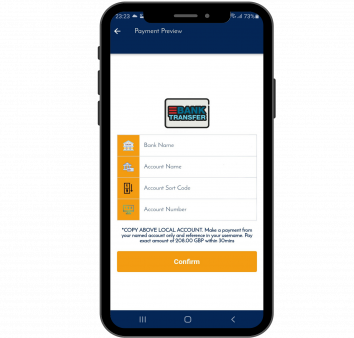The image features a detailed outline of a cell phone interface. On the left side, there are three grey buttons: the top one is small, while the two underneath it are of equal length and the rightmost one is slightly longer. The interface has a black outline, and in the top left corner, there's a small, illegible white text.

A blue box area contains white font and a left-pointing white arrow with the label "Payment Preview" beside it. Below this section is a white box area with black outlines and text in red and powder blue that appears to read "Bank Transfer." A red box is situated next to this text.

On the next line, there are four grey boxes with faint grey font. An orange box displays similarly faint images and grey text on its left. Beneath these elements, there's unreadable grey text, followed by the words "Local Account," with the rest of the text being too small to discern.

Centered below is an orange square with "Confirm" written in white font. The white box area terminates, and at the very bottom, within a blue box, a slight white font extends from left to right, described as three vertical white lines, a white square, and an ambiguous white shape that resembles either a 'C,' an 'E,' or a phone.